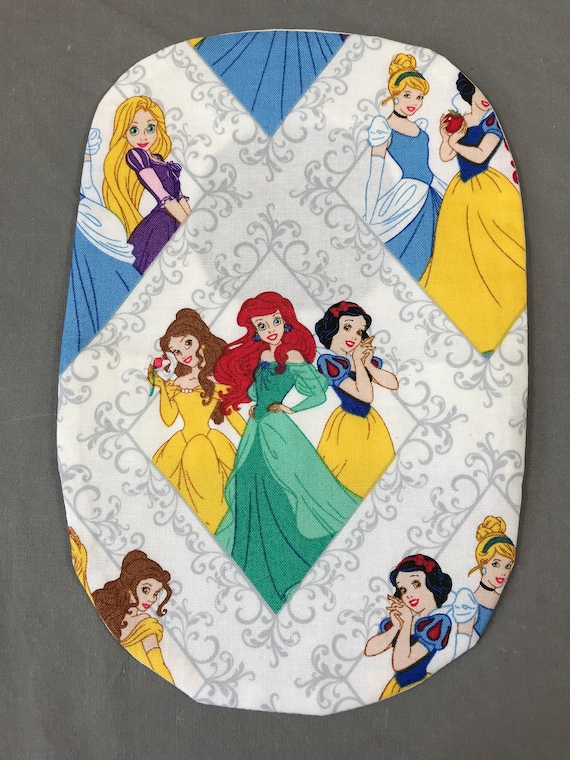The image displays an oval-shaped object with an irregular outline. It is adorned with a decorative fabric that has a white base featuring curling gray patterns. Interspersed within these patterns are diamond-shaped frames, each containing illustrations of Disney princesses. Prominently featured in the center are cartoon depictions of Belle in her yellow gown, Ariel (the Little Mermaid) in her iconic green dress, and Snow White in her traditional dress, all captured in various poses. Additional frames showcase Cinderella and Rapunzel, the latter dressed in her signature purple attire. The entire composition is set against a gray background, giving the object a whimsical and enchanting appearance.